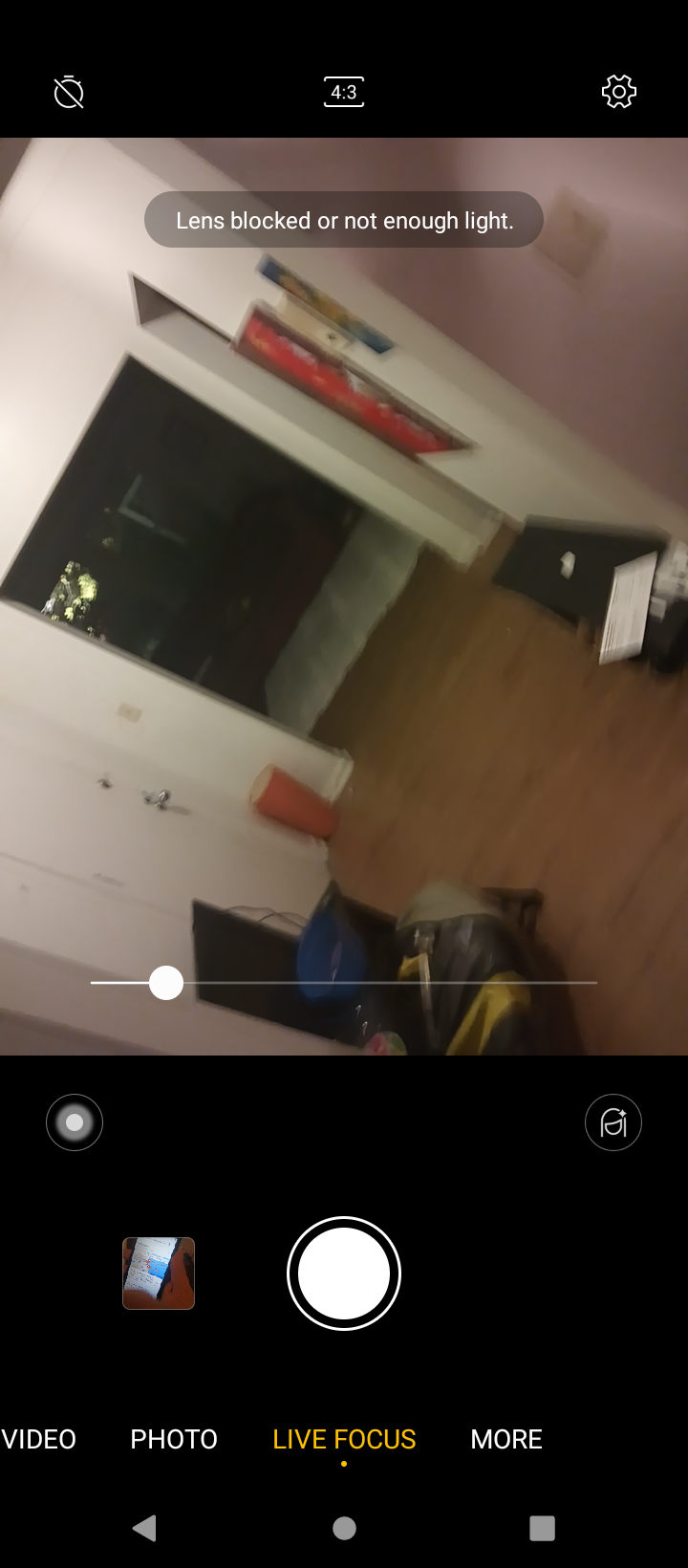This image, captured on a smartphone, is somewhat obscured by a warning indicating either a blocked lens or insufficient lighting, resulting in a limited field of view. The scene appears to be taken from an elevated vantage point, possibly a staircase, providing a partial overlook into a room with wood flooring. This room seamlessly transitions into a larger adjoining space adorned with a rug over its wooden floor.

On the left side of the larger room, a window—potentially a picture window—offers a glimpse of the exterior, though its specifics are not clear. The wall closest to the camera is painted a mauve color, which contrasts with the predominantly white walls of the larger room. An orange, narrow trash can is positioned in the corner to the left.

On the floor near this trash can, there's an open device, accompanied by what seems to be an electronic robot designed for automated tasks. Despite the limited visibility, the photo captures a blend of minimalist decor and functional electronic elements, all under subdued lighting conditions.